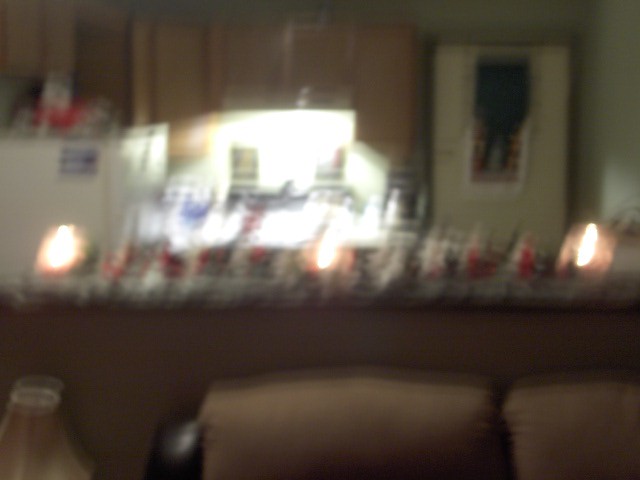In this slightly blurry photograph, the foreground reveals a partial view of a tan and brown couch, accompanied by a fragment of an off-white lampshade to its side. Behind this couch, a kitchen countertop stretches across the backdrop, presenting a blend of tan, brown, and white hues. Resting on this counter are a few red and white objects, alongside what seem to be two candles with perceptible flame outlines. An overhead light casts an illuminating glow on orange-blonde cabinets that line the kitchen space. To one side of the image, a white refrigerator stands adorned with a few blue magnets and topped with additional red and white items. The overall scene is softly lit, contributing to the cozy ambiance despite the blur.